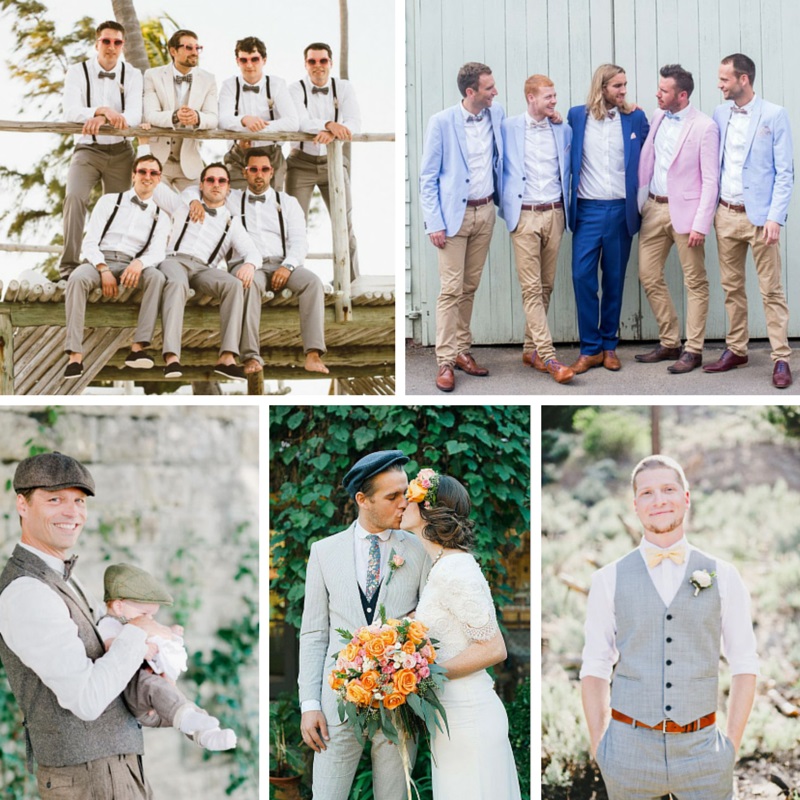This collage appears to be part of a photo album from a wedding, featuring five distinct pictures arranged in a mosaic. The top row consists of two images: the left one shows seven groomsmen dressed in grey pants, white shirts, grey bow ties, and round sunglasses, with suspender belts; they are seated on a structure that resembles a beach house shade. The right image displays five friends in suits, hugging and smiling, with the groom prominently in the center wearing a navy suit.

The bottom row contains three pictures. On the left, a man in a grey monkey jacket and brown pants is seen holding a baby. The middle photo captures a tender moment between a bride and groom; she is in a white wedding gown, holding a bouquet of orange, peach, and pink flowers, and he is in a grey suit with a colorful floral tie. The final image on the bottom right features a man posing in a natural setting, dressed in a grey vest, grey pants, white shirt, and yellow bow tie. The collage prominently features colors like grey, white, brown, blue, orange, pink, beige, black, and green.